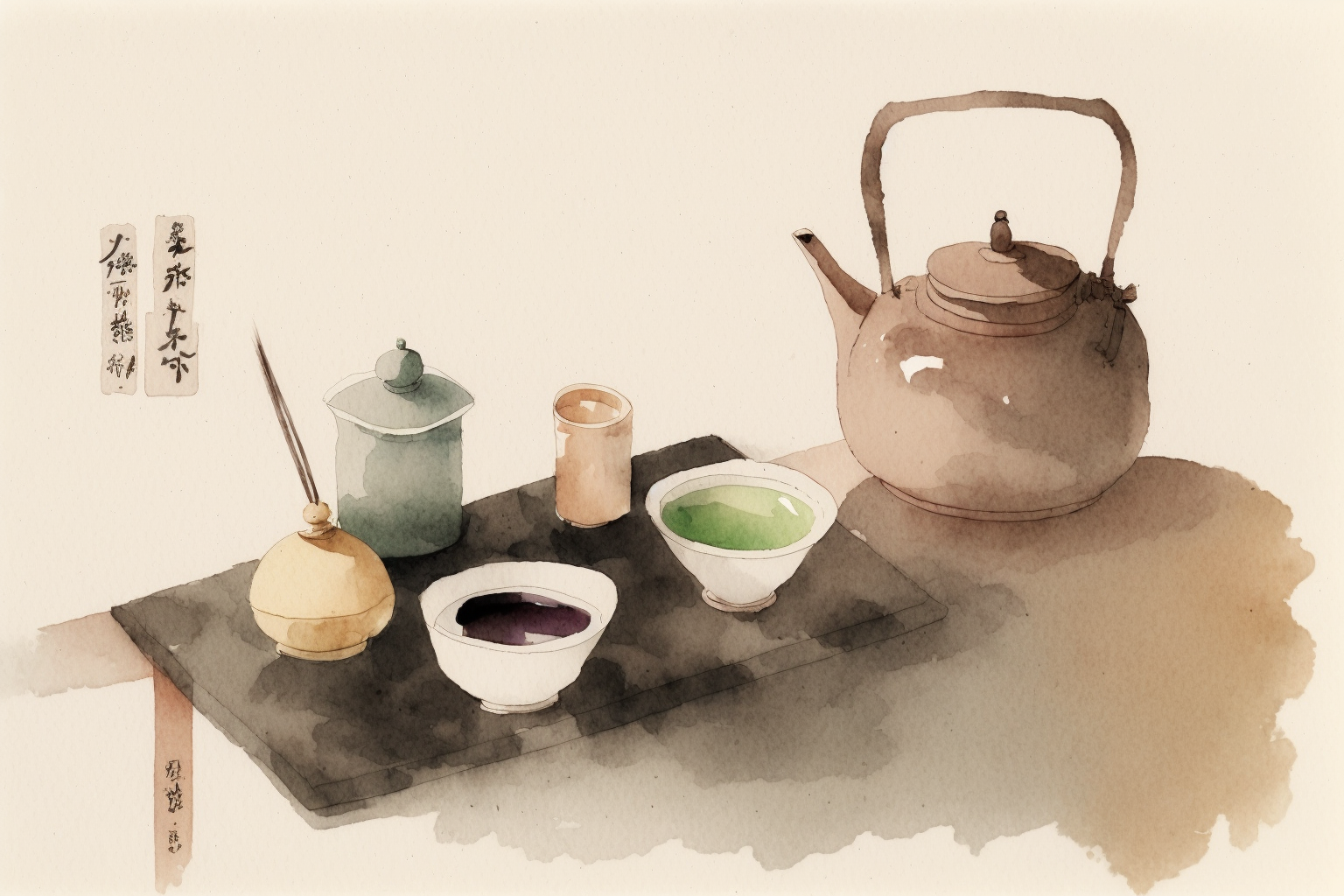A watercolour painting features a detailed yet dreamy tea set arrangement, evoking a Japanese artistic style. On the far left, vertical strips of paper with black Kanji writing provide cultural context. The central focus is a tan teapot with a curved handle and a spout on the left side, crowned by a small cap. It sits atop a table that appears fluid and unfinished in the watercolor technique. To the right of the teapot, a black rectangular surface adds contrast, functioning either as a mat or a tray. This dark surface holds two white bowls, one with a green liquid and the other with a black-brown liquid. Joining them are three distinct containers: a peachy-brown cylindrical glass, a round cream-colored vessel with a cover and an inserted pen-like object, and a blue vase with a cap. The harmonious blend of tan, gray, and black tones with the fluid lines and soft edges create a serene, almost ethereal representation of a traditional tea set.